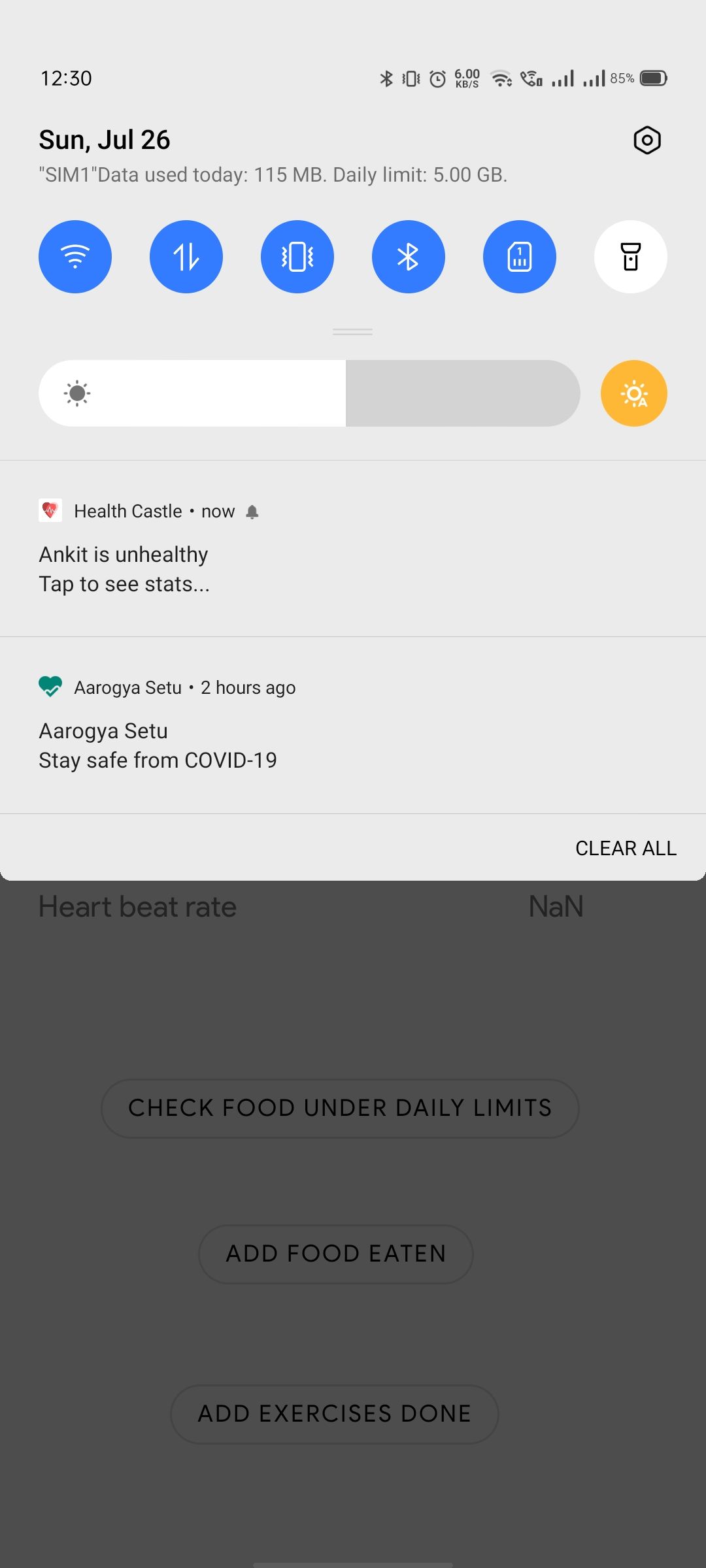Here is a cleaned-up and detailed caption for the image described:

---

A screenshot captured from a cellphone displays a user interface with a gradient background that transitions from light gray at the top to darker gray at the bottom. At the top, the date "Sunday, July 26th" is visible, alongside data usage details indicating "SMI data used today: 115 MB" with a daily limit of "5.0 GB." Beneath this text are five blue icons followed by a white icon resembling a trash can. The brightness setting is also shown, adjusted to slightly above the halfway mark, with an orange circle at the end of the brightness control slider. Further down, under the "Health Castle" section, a notification reads: "Ankit is unhealthy. Tap to see stats." Continuing down, a green heart icon appears next to the text: "Araghar set to 2 hours ago. Araghar set to stay safe from COVID-19." The bottom of the screen is less legible due to the darker gray shading in that area.